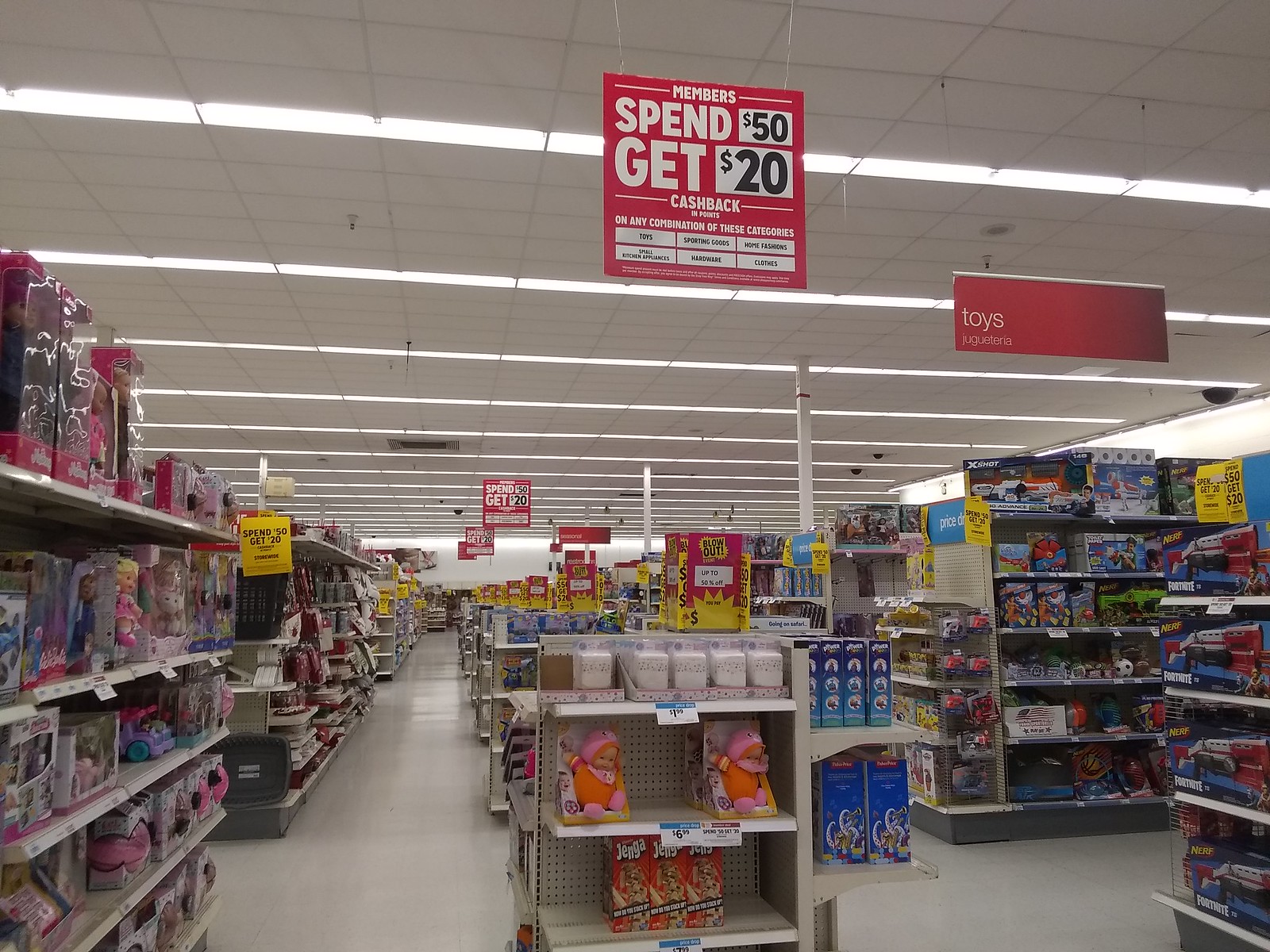In this rectangular photograph, we find ourselves in the aisle of a store, specifically in the bustling toy department, surrounded by numerous sale items. On the left-hand side, an end cap displays a selection of dolls, girls' helmets, and pink and purple toy cars, all neatly arranged to catch the eye. Moving our gaze to the right, a three-tiered center display stands prominently. On the bottom shelf of this display, the game Jenga is available for $17.99. The middle shelf features small baby dolls in vibrant orange and pink, each priced at $6.99. At the very top, there’s a square item priced at $1.99, although the specific nature of this item remains unclear. Continuing to the right, another end cap showcases an array of Nerf guns, specifically branded with the Fortnite logo in the lower left-hand corner. One particular aisle is lined with a diverse range of toys and games, including various Nerf products. At the bottom of this aisle, we can see a basketball hoop set paired with a Nerf ball, adding a sporty option to the extensive selection of toys. The image captures the lively and colorful atmosphere of the toy department, emphasizing the variety and excitement of the available products.